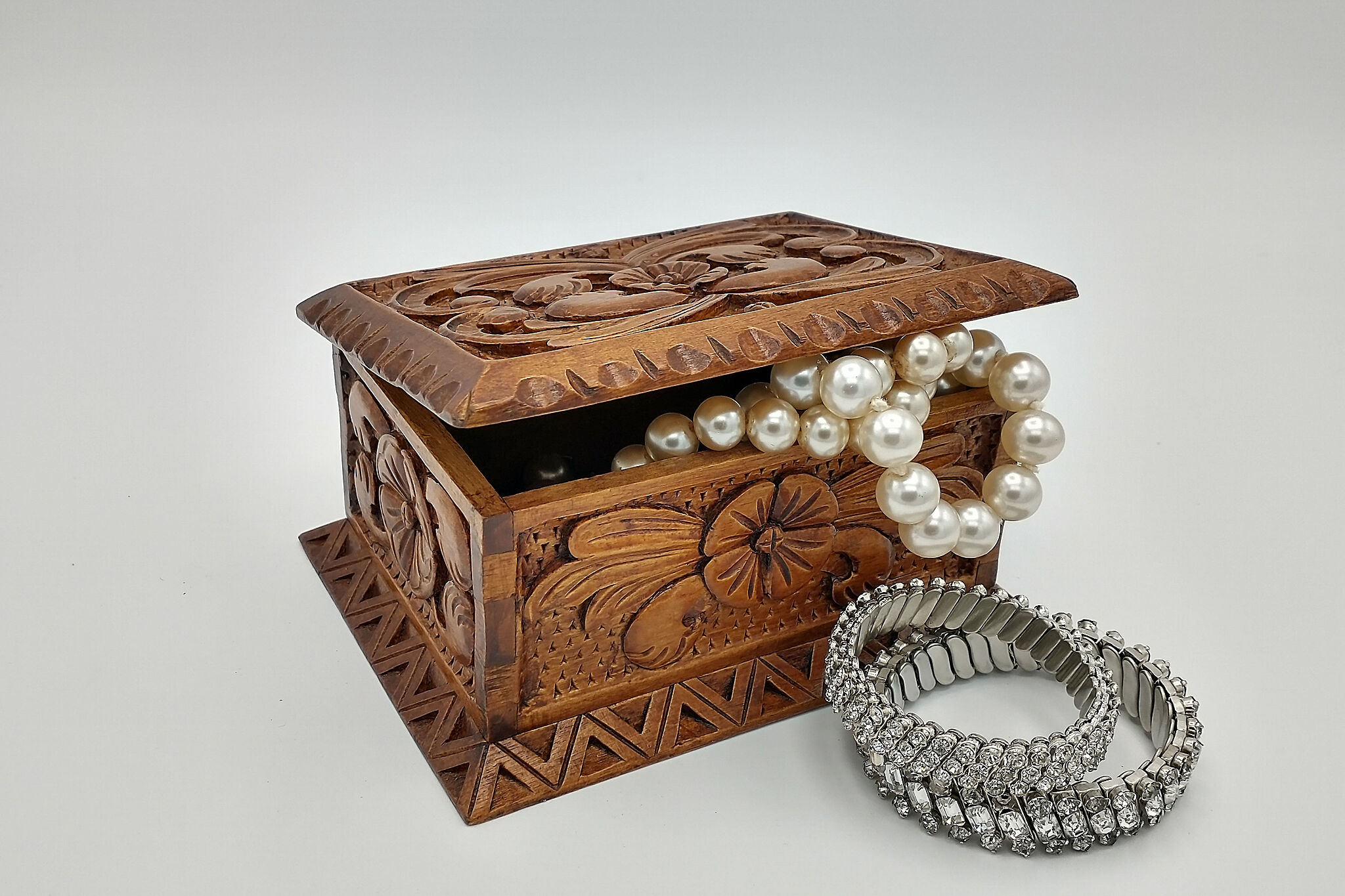The image depicts an exquisitely ornate wooden jewelry box, featuring intricate hand-carved floral designs on its lid and sides. The base showcases a geometric triangle pattern that frames the box. The finish is a rich, dark brown, enhancing its handcrafted appeal. The box is slightly ajar, with a golden pearl necklace draped over the lip, preventing the lid from closing completely. This adds a delicate touch to the overall composition. Positioned beside the jewelry box are two elegant silver crystal bracelets, contributing to the decorative ambiance of the scene.